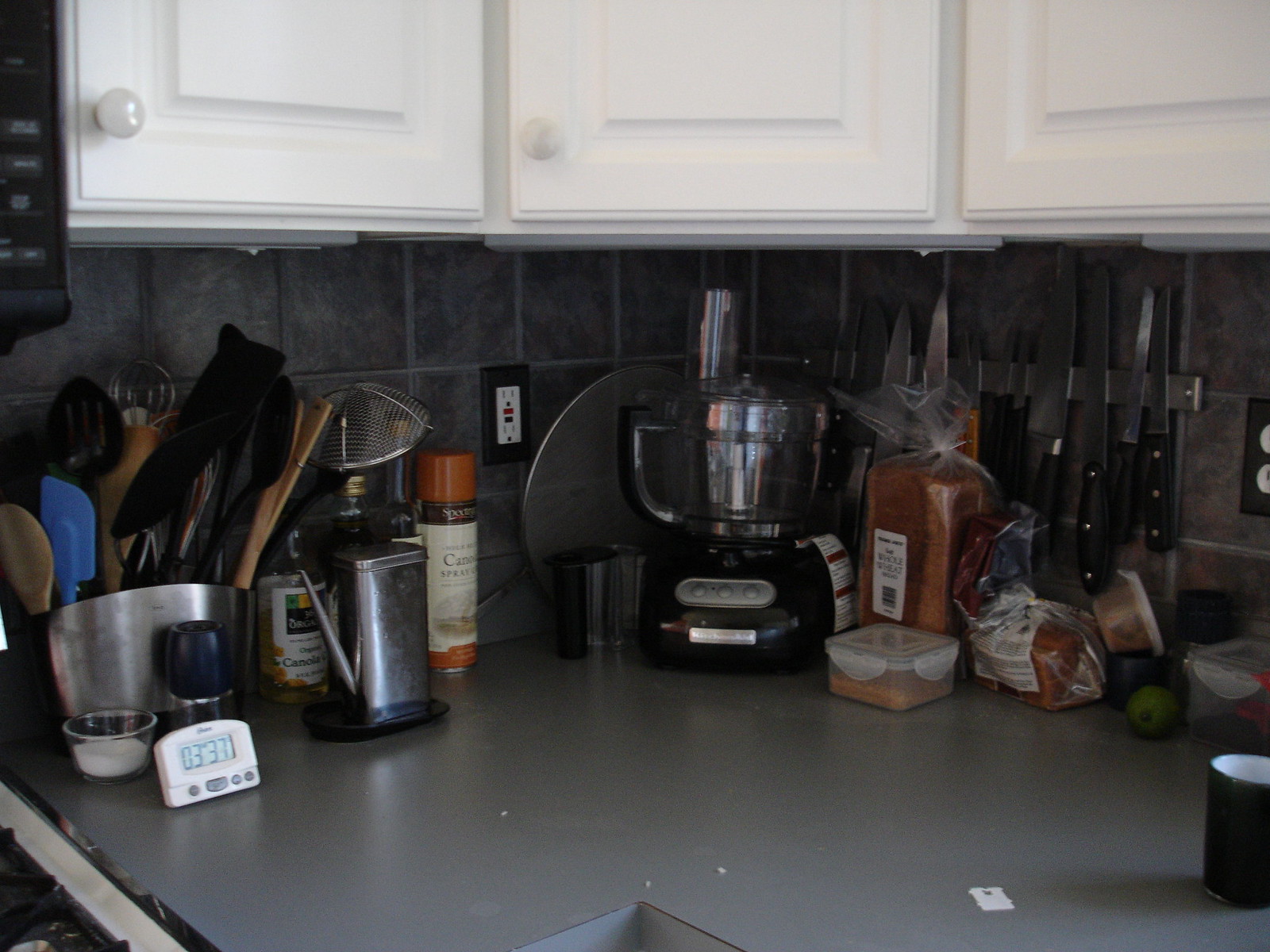The photograph captures a cluttered kitchen counter situated in a corner, revealing a textured subway tile backsplash that is not white. Above the counter, a set of white corner cabinets with wood inlays and round knobs is visible, though the under-cabinet lighting is turned off. The gray countertop in the corner is adorned with various items. 

In the foreground, a small white timer with indistinguishable numbers is positioned near a clear, round dish containing salt. Behind these, a stainless steel bowl is brimming with an assortment of cooking utensils, including spatulas and wooden tools. Adjacent to the utensil bowl, a Lazy Susan holds a collection of items, including a bottle of olive oil and a stainless steel container, possibly for spices. 

An electrical outlet is situated on the backsplash. Turning the corner of the counter, there is a blender rather than a coffee pot. Nearby, several bottles, a small plastic container with unidentified contents, a bag, a bread tie, and a coffee cup contribute to the cluttered scene.